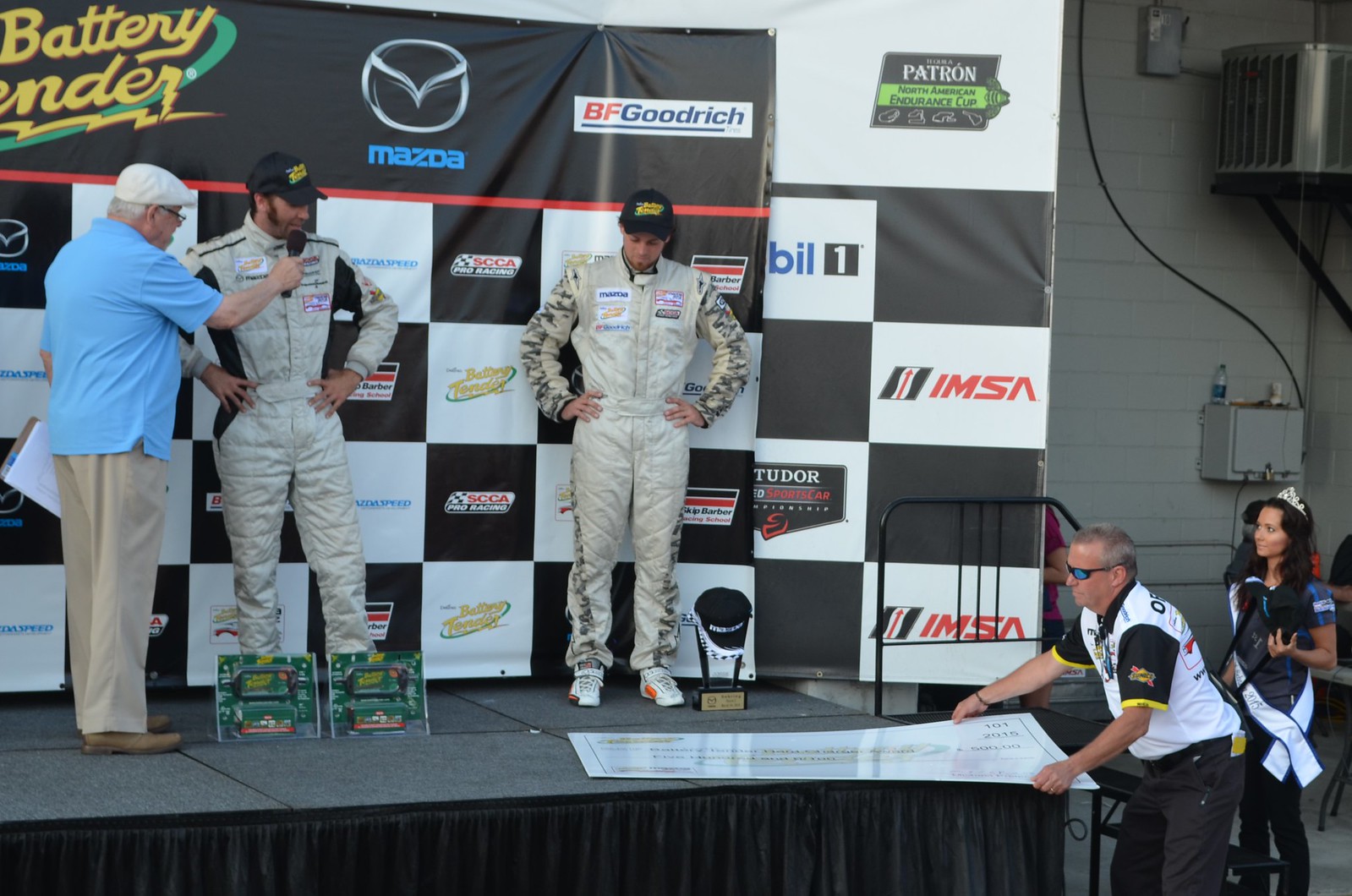The image features two men wearing white, one-piece cow-raising uniforms standing on a stage, each sporting black baseball caps with yellow logos. The man on the left has black lines on his uniform, while the man on the right has gray patterns on both arms. To the far left, another man, appearing elderly with gray hair and glasses, holds a microphone in front of the man on the left. This man is dressed in a blue short-sleeved polo shirt, beige pants, brown shoes, and a white cap. In the background, a black and white checkered banner with multiple business logos, including 'Master' and 'BF Goodrich', is displayed. The stage itself has a black curtain along the bottom part and is set against a backdrop of grey cinder block walls, visible behind the banners, with air conditioning units and electrical boxes mounted on them.